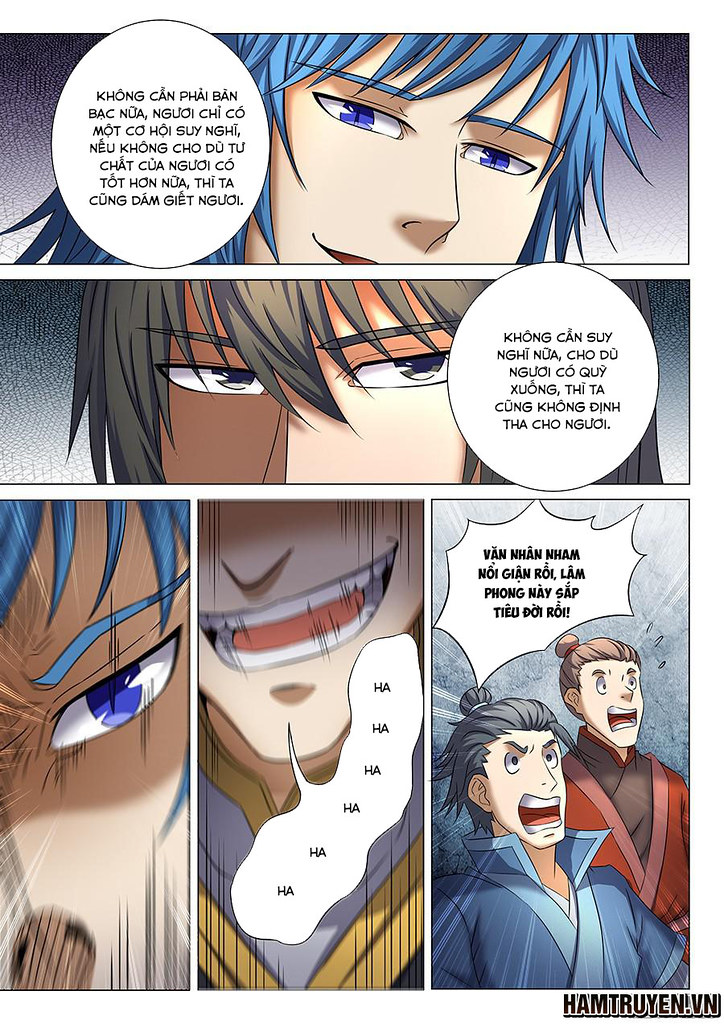This image is a vertical rectangular comic strip styled in an anime fashion, consisting of five distinct panels. The top two panels are arranged horizontally, while the bottom three panels are vertical, positioned directly beneath the horizontal ones. There are three central characters, possibly four. 

The first panel at the top features a character with blue hair and blue eyes, accompanied by a large speech balloon containing text in an unknown language. Below this, the second horizontal panel showcases another character with dark hair and dark eyes, half of her face is brown and the other half is white, and she also has a speech balloon. 

In the vertical sequence below, the first panel is a close-up of the blue-haired, blue-eyed character. The next vertical panel focuses on a close-up of a mouth with a speech balloon containing the repetitive text, "ha ha ha ha ha," depicting an evil laugh. The final vertical panel shows two other characters with expressions of shock on their faces.

Additional details include some text at the bottom right corner of the entire strip, spelling out "H-A-M-T-R-U-Y-E-N!" followed by "V-N." The text in the speech balloons appears to be in a non-English script, potentially a South Asian language. The overall style and themes suggest it might appeal to teenagers.